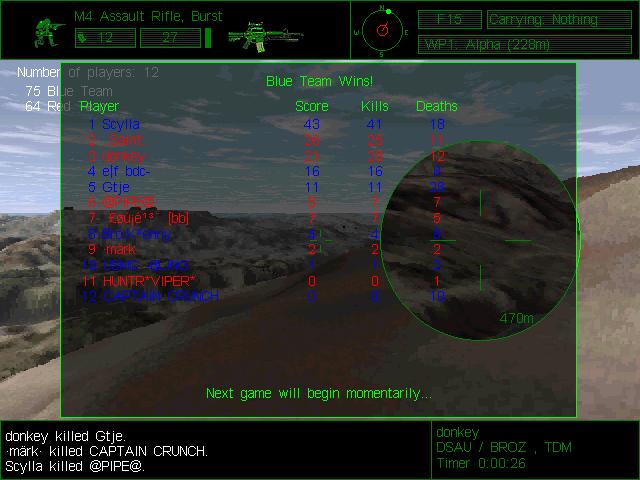This video game screen capture showcases a barren, rocky landscape, evocative of a desert terrain. Central to the image is a crouched military figure armed with an M4 assault rifle, detailed beside him. Positioned atop the screen, a black bar features green text and numerical data—highlighting specifics like the armed soldier's M4 burst mode with a count of 12 and the code 27.

Adjacent on the right of this bar is a compass icon, indicating a direction slightly right of north, coupled with labels such as F15, carrying nothing, WP1 Alpha, and a distance notation of 228 meters. Centrally overlaying the image is a semi-transparent gray panel listing player statistics, although some names and numbers are blurred. Clear entries include Skilla with a score of 43 (41 kills and 18 deaths), Elf BDC with a score of 16 (16 kills and 8 deaths), and GTJE with 11 points (11 kills and 28 deaths). An inset within this panel displays a zoomed-in view of the terrain with a gun sight, marking a target 470 meters away, accompanied by a notification that the next game will commence shortly.

The bottom of the screen features another dark banner, listing recent in-game events in green text on the right, such as "donkey DSAU/BROZTDM timer 0:00:26". On the left, it records combat updates like "donkey killed GTJE," "Mark killed Captain Crunch," and "Skilla killed at pipe at."